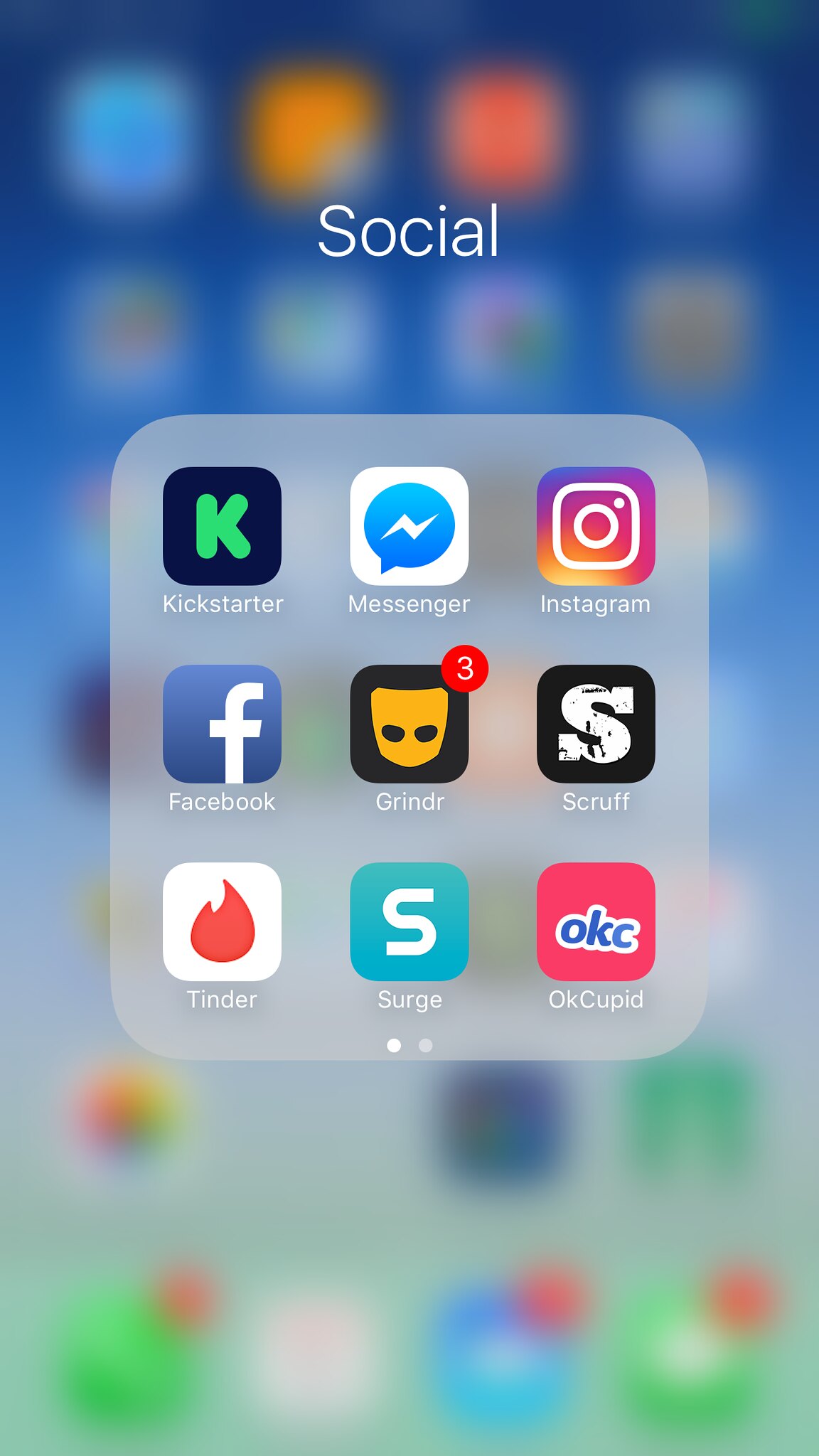A detailed screenshot captures the home screen of a smartphone, specifically focusing on the "Social" category. The image is in portrait orientation, and the entire background has been blurred to highlight content in the foreground. At the top center, the word "social" is prominently displayed in a thin, white font.

Centrally positioned is a slightly translucent gray square with rounded corners. Within this square, a 3x3 grid showcases various app icons categorized under social media and dating. From left to right and top to bottom, the displayed apps are:

1. Kickstarter - featuring a black background with a prominent green "K".
2. Messenger - a white square adorned with a blue thought bubble containing an electric loop.
3. Instagram - recognizable by its vibrant multicolored camera logo.
4. Facebook - identifiable by its blue square and white lowercase "f".
5. Grindr - with its distinctive yellow mask-like icon.
6. Scruff - easily spotted with its orange background and mascot dog design.
7. Tinder - marked by its red flame logo.
8. Surge - showcasing a blue gradient square with a white swirl design.
9. OkCupid - recognized by its blue text "OKCUPID" on a pink and blue gradient background.

Below the 3x3 grid, two navigation dots indicate the presence of multiple app pages. The left dot is highlighted, signifying the current page, while the right dot remains grayed out.

Overall, the precise arrangement and clear visual cues in the image present a structured overview of the user's social apps on their smartphone.